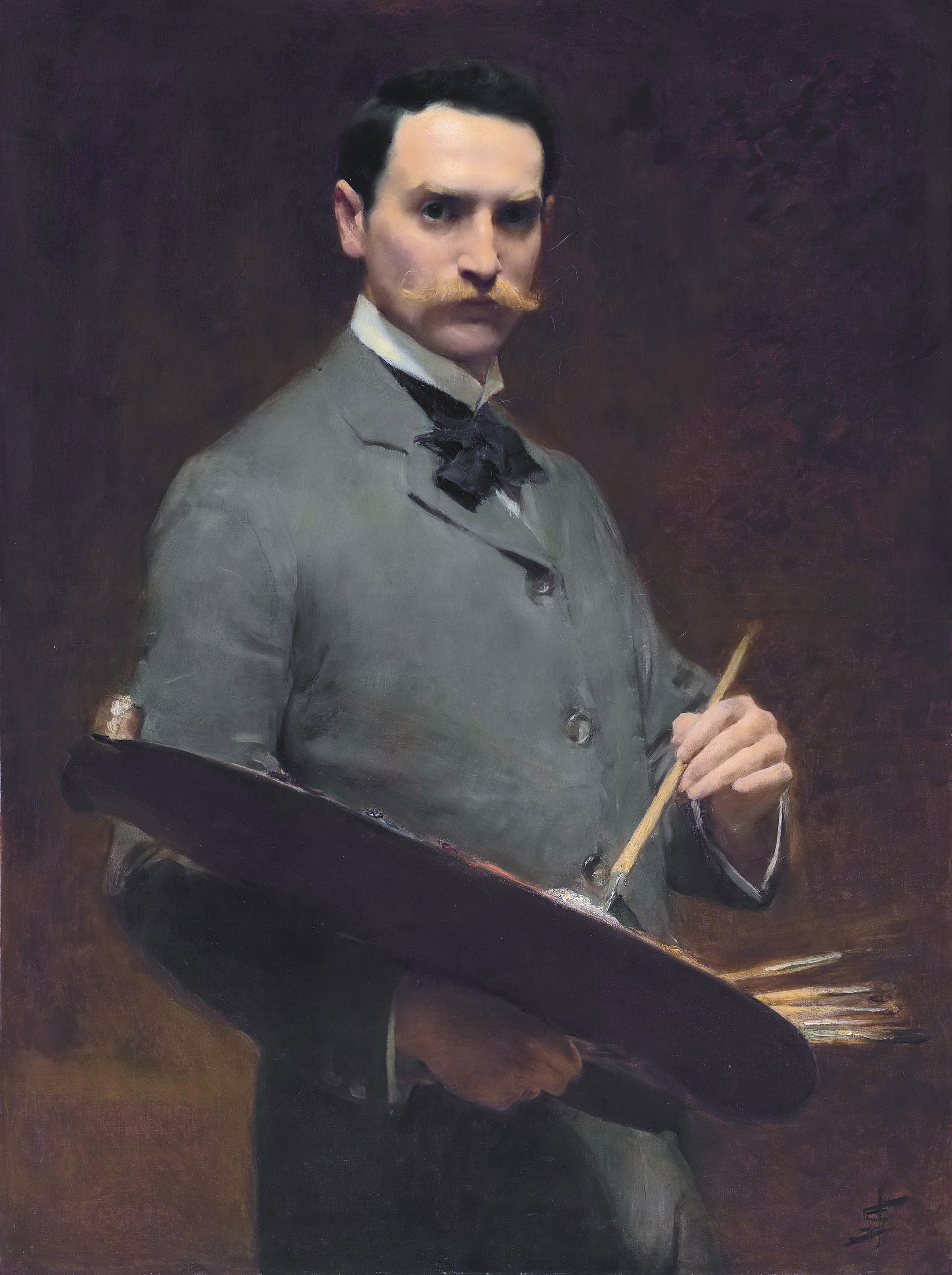The image portrays a striking self-portrait of an artist, likely in his thirties, characterized by his stern expression and dramatic lighting that accentuates his features. He is centrally positioned in the painting, dressed in a classic, gray button-up jacket with a vintage, thick black tie reminiscent of the 1800s. The man has short, dark hair and a wide, blonde handlebar mustache. In his right hand, he holds a painter's palette, while his left hand holds a brush resting on the palette, indicating he is in the act of painting. The overall color palette includes shades of gray, white, black, and brown, contributing to the painting's vintage aesthetic, possibly dating back to the 1930s or 1940s. Behind him, although not visible, he is presumably engaged with a canvas. The meticulous details suggest the work of a talented and possibly renowned artist, showcasing his remarkable ability through this evocative self-portrait.